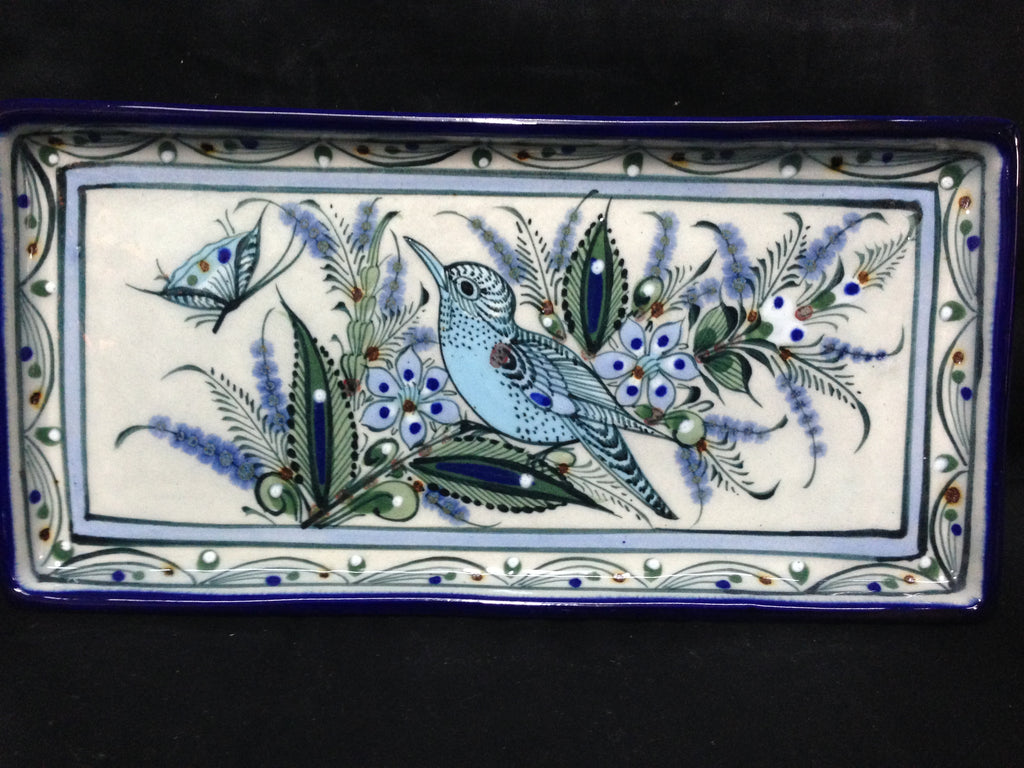This detailed color photograph depicts a small, rectangular porcelain serving dish, likely glazed ceramic, resting on a black surface. The focal point of the dish is a beautiful light blue bird with a cool blue design on its wing and a distinct black eye. The bird is perched on a branch adorned with peacock-like blue flowers and green leaves. Surrounding the central image, an intricate pattern includes a small blue and black butterfly with three notable dots—blue, red, and green—on its mostly white wings. The central design is framed by a light blue square border, accentuated by delicate motifs resembling shimmering lights. The dish's overall appearance is elegant and intricate, featuring a combination of dark blue and white backgrounds that highlight the vivid decorative elements, making it suitable for display rather than daily use.